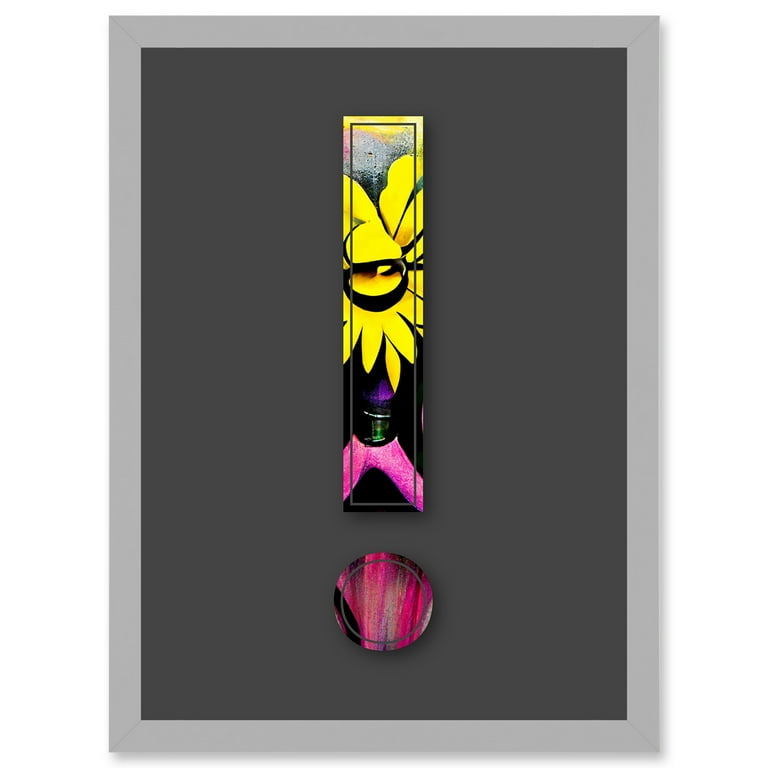The image showcases a vibrant and whimsical piece of artwork that features a large rectangular frame. The outer border of the rectangle is gray, with a dark gray interior. At the center of this rectangle, there is a painting of a yellow flower-like object that is suggestive of a lamp, with black detailing resembling a tube extending downward. Attached to this tube is a hot pink, almost fuchsia, stand or base. Below this rectangular piece is a separate, round object that resembles a coaster or a decorative wooden circle with hot pink brush strokes, adding a playful touch. This round piece further complements the exclamation-point-like visual arrangement of the artwork. The entire scene is set against a dark gray background, which is bordered by a gray frame that enhances the vibrancy of the other colors, creating a striking and coherent display.